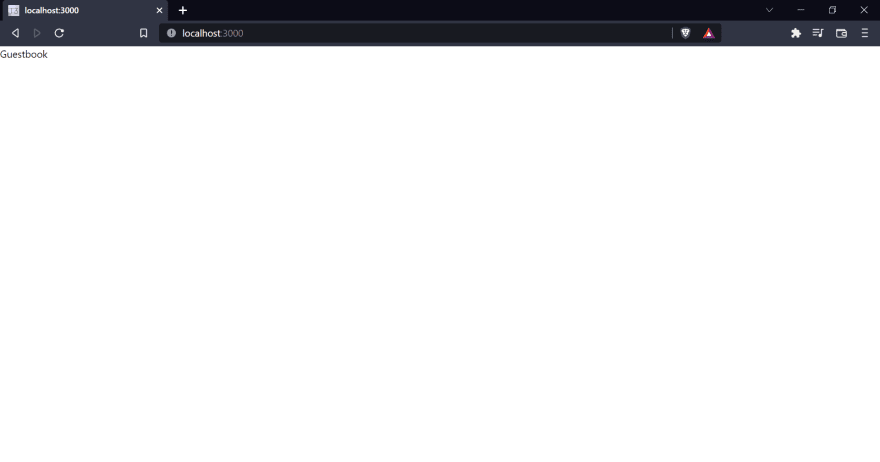A detailed caption for the image:

"The image captures a website displayed within a minimized Google Chrome browser window on a Windows operating system. The browser appears to be in dark mode, evident from the black taskbar and dark interface elements. In the upper right corner of the browser window, icons for closing (X), maximizing (two overlapping squares), and minimizing (a dash) are visible. The address bar reads 'localhost:3000' and has several icons, including a puzzle piece indicating extensions and a red triangle likely representing a notification or alert. Other visible icons include a book icon, a refresh button, a forward arrow (grayed out), and a back arrow. The webpage itself displays the text 'guestbook' in small font, while the rest of the page is blank white, suggesting that the content has not loaded properly. The overall impression is of a local web page in development or a malfunctioning site with only the address 'localhost:3000' and the text 'guestbook' rendering correctly against a white backdrop."